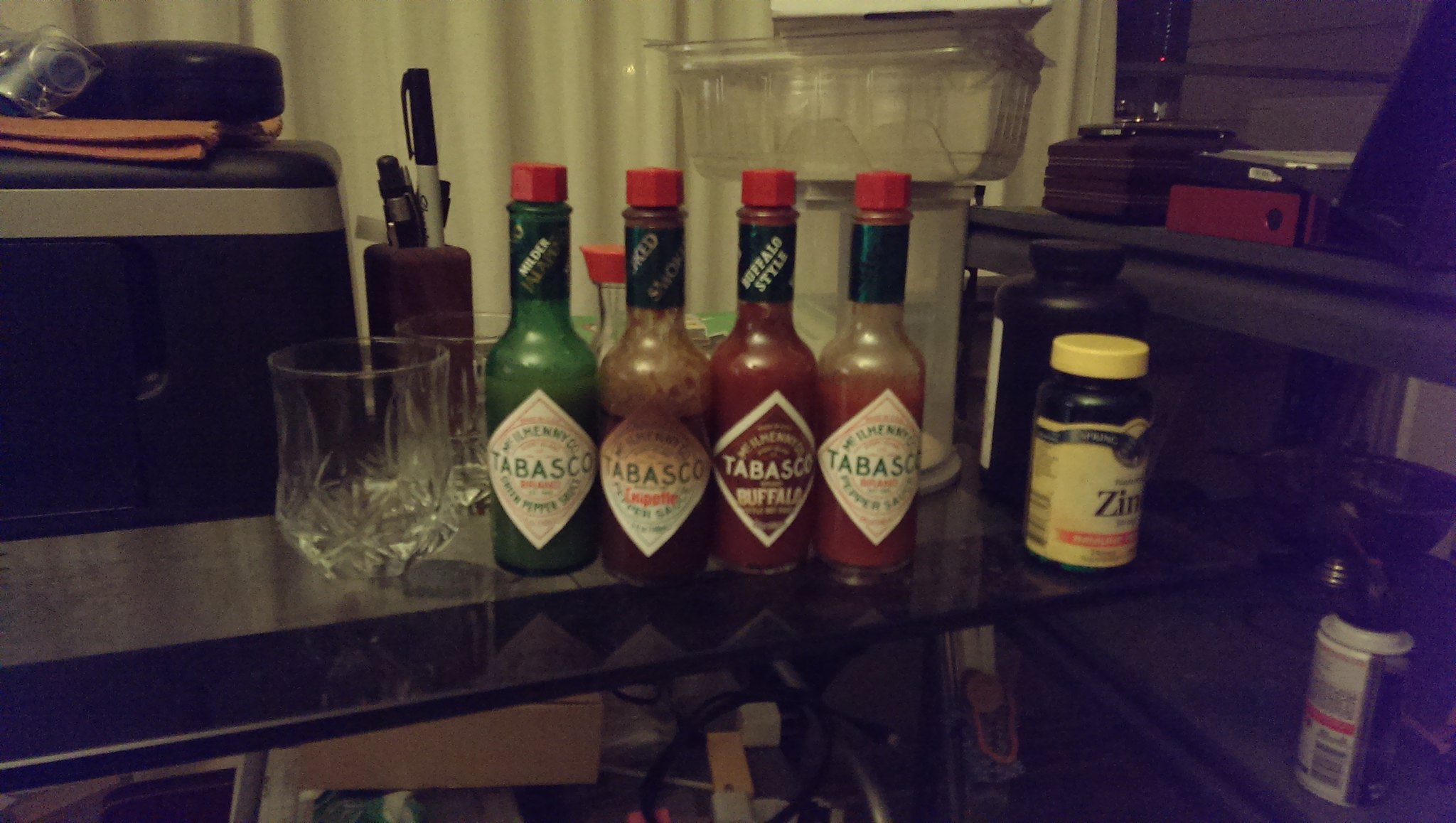In a somewhat dimly lit, landscape-oriented photo with a yellowish tint, a small collection of Tabasco sauce bottles takes center stage on a flat, reflective surface, possibly a glassy bar or kitchen bench. There are four distinctive bottles lined up front and center, each with a red lid. From left to right, the first bottle contains green Tabasco sauce, the second is an older, dark brown bottle with noticeable use, the third is a full Tabasco buffalo sauce with red contents, and the fourth is a partially used bottle of traditional red Tabasco sauce. To the left of these bottles sit two empty tumbler glasses. To the right, there is a bottle that appears to be zinc supplements or vitamins. The background remains ambiguous, featuring unidentifiable objects that could include containers, a cylindrical wooden pen holder with markers, a potentially corrugated white curtain, and possibly a shelf with various items. The overall scene is intriguing, albeit cluttered, with the main focus unmistakably on the array of Tabasco sauces.